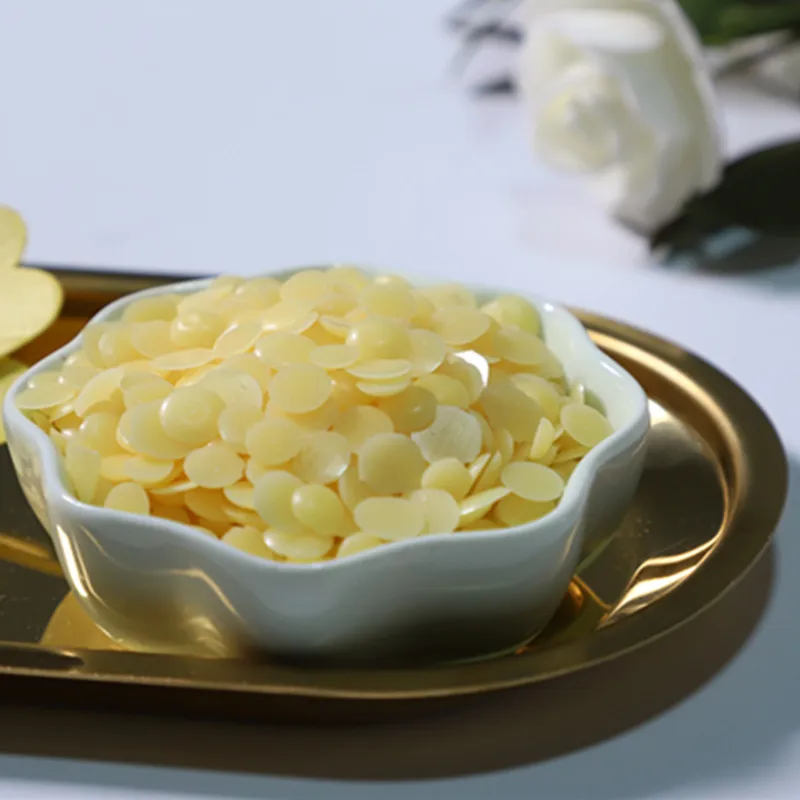In a stark, minimalist setting, the photograph captures a serene arrangement atop a white table. At the forefront is a white, flower-shaped porcelain bowl with scalloped edges, exuding a glossy shine. This bowl is filled with numerous thin, flat, yellow butter-colored wax melts, arranged in circular discs that evoke the appearance of delicate potpourri. The bowl is placed on an oval, shiny brass platter, which subtly reflects both the bowl and its contents, creating intricate shadows on the table surface. To the left of the porcelain bowl, partially out of frame, resides a smaller yellow dish, also resembling a flower. The background blurs gently, featuring a white rose with visible green leaves on the right-hand side, lending a touch of natural elegance to the composition.